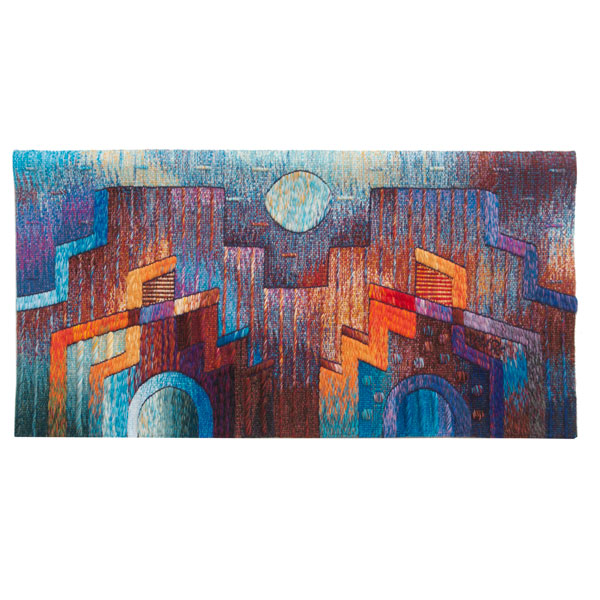This abstract drawing depicts an imaginative cityscape, characterized by geometric and angular shapes that hint at buildings under a faintly visible sky and a central, large white circle resembling a moon adorned with subtle eye-like symbols and swirling hints of orange and blue. The scene features a rough, textured mix of colors—bright turquoise, light blue, brown, orange, yellow, and purple—that are applied vertically in a messy, layered fashion. Dominating the foreground, two symmetrical structures stand with rectangular tops and staircase-like sides, each with a large circle in front of their doors. The left circle displays thin vertical lines within a blue and yellowish hue. The right circle has a bluish-purple shade with a centered blue hue, dotted with smaller circles. The bottom center is predominantly brown, while the upper areas transition to vivid blues, creating a stark contrast with the polka dot and striped patterns that embellish the abstract buildings. A white line flanks either side of the moon-like circle, adding to the composition's depth and whimsy.